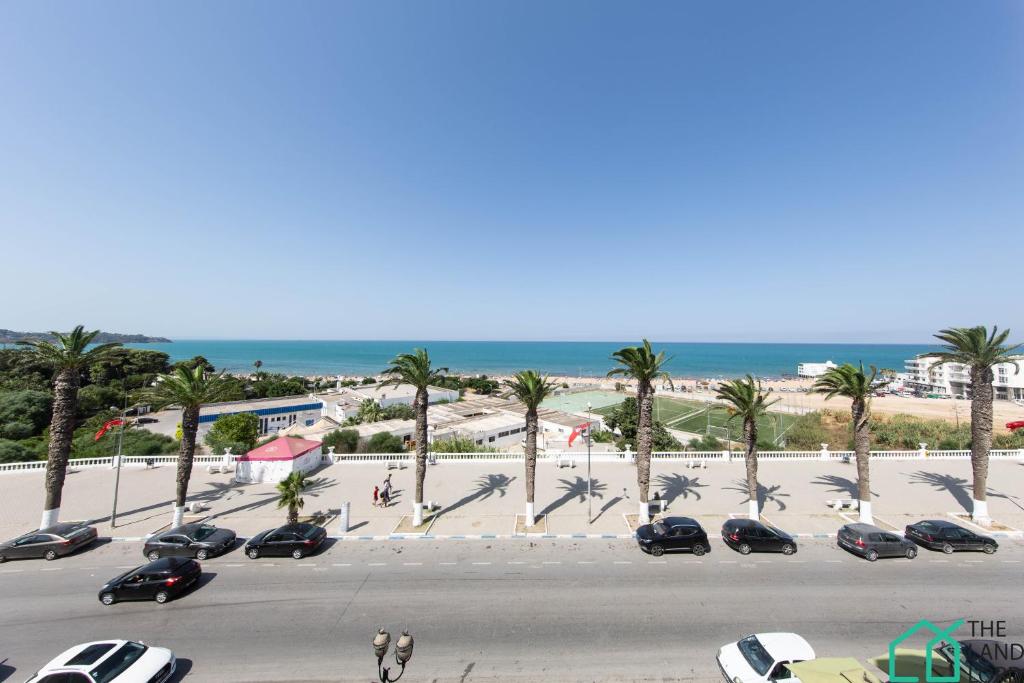The image captures a vibrant, picturesque beach town, likely a resort area, on a beautifully clear day with a bright blue sky. In the foreground, a cement road runs horizontally, flanked by parallel-parked cars on either side. One car is actively driving down the street. Adjacent to the road are lampposts or meters, and on one side, there's a small outhouse with a red roof and white walls. Beyond the road, a broad sidewalk can be seen, along with a railing that overlooks the surrounding structures— a mix of houses and buildings.

There is an array of palm trees lining the boulevard in front of the beach, numbering about eight, which adds to the tropical ambiance. Further into the scene, the image reveals a green space, possibly a tennis court or similar recreational area, leading to the sandy beach dotted with people. The beach itself stretches horizontally from the left, where trees are visible, to the right, where several white buildings stand.

In the background, there are additional white-and-blue striped buildings and residential structures. The scene is set against the dark blue waters of the ocean, which meets the clear sky on the horizon, creating a seamless blend of colors. The overall composition, enhanced by the cloudless, brilliant blue sky, showcases the serene, inviting atmosphere of this beachside community.